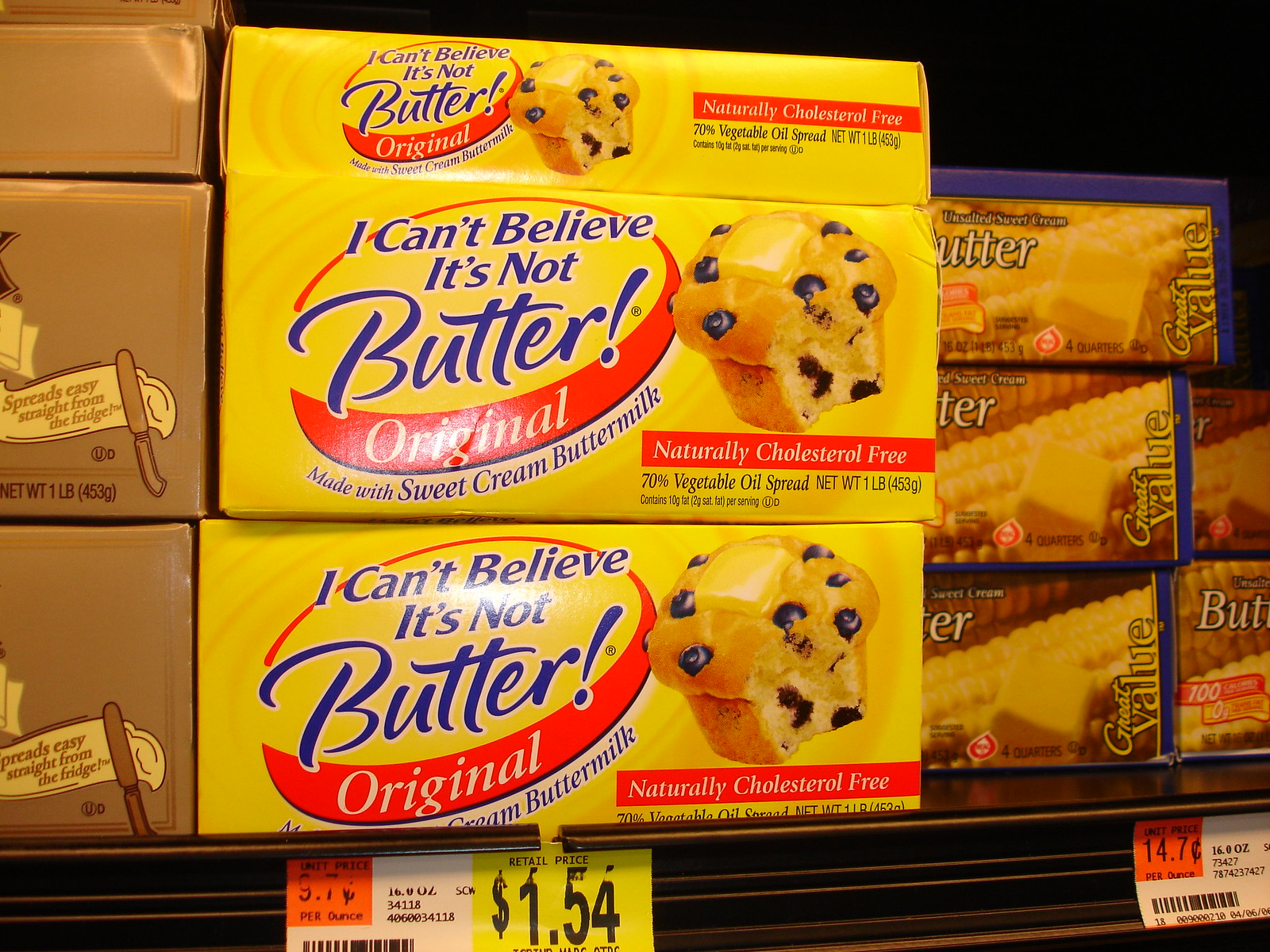This detailed photograph captures a grocery store shelf displaying various butter products. In the center, the focus is on three stacked yellow containers of "I Can't Believe It's Not Butter! Original," each adorned with a blueberry muffin image and blue writing. Notably, the packaging mentions it's made with sweet cream buttermilk and is naturally cholesterol-free. These containers are priced at $1.54 each, as indicated by the retail labels at the bottom of the image. To the left of these containers, there is a gold-packaged butter product featuring an image of butter being spread with a knife, though the brand name is not visible. On the right, there is another butter product in unsalted sweet cream butter packaging, labeled with a piece of corn in its design and marked with the "Great Value" brand. The setting clearly depicts a typical well-organized aisle in a grocery store.